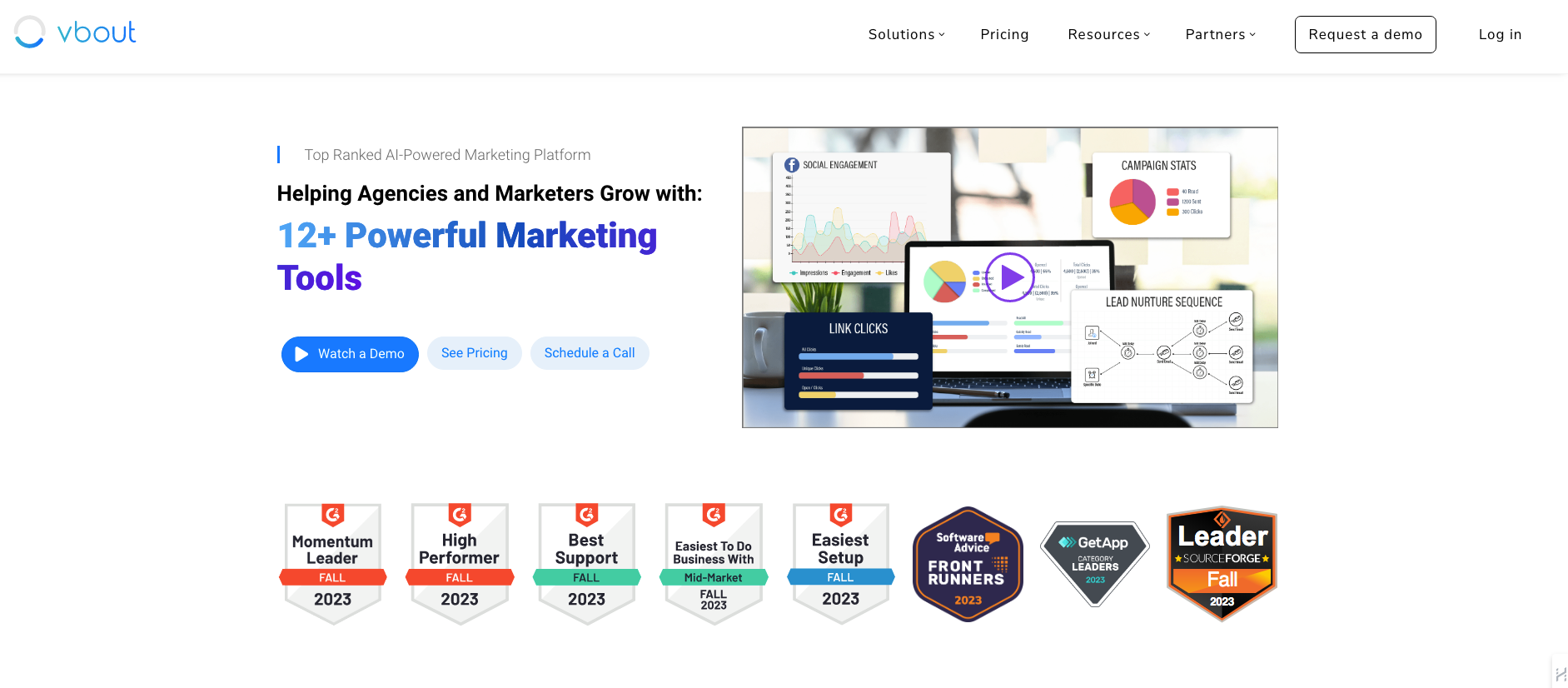An advertisement for VBout, a premier AI-powered marketing platform, is displayed prominently on a web page. The top of the page features a striking headline in blue gradient text that reads, "12+ Powerful Marketing Tools." Just above this, a smaller caption in black emphasizes, "Helping agencies and marketers grow with 12+ powerful marketing tools." 

In the upper left corner, the company name, VBout, is clearly displayed. The navigation menu offers quick access to sections such as Solutions, Pricing, Resources, Partners, Request a Demo, and Login.

The main visual element showcases an array of computer screens displaying various marketing tools, hinting at the platform's comprehensive capabilities. Below this visual, the platform proudly displays its numerous accolades, including titles such as Momentum Leader, High Performer, Best Support, Easiest to Do Business With, and Easiest Setup from a leading magazine. Additional recognitions from software review platforms like Software Advice, FrontRunners, GetApp, and Leader further underline VBout's industry-leading status.